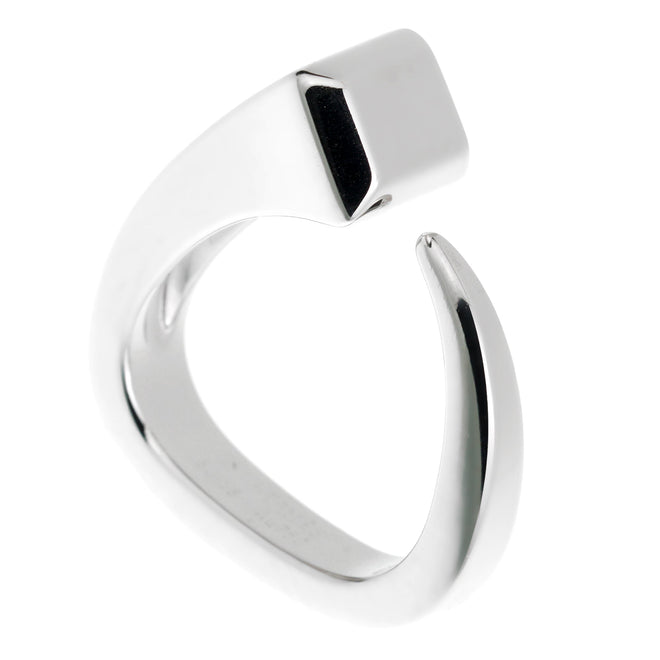This is a highly detailed and large photograph of an abstract metal ring, set against a completely white background. The ring is made of a shiny, reflective material, likely silver, white gold, or stainless steel, making it difficult to distinguish the exact metal type due to the lighting. The ring features an incomplete circular shape, reminiscent of an upside-right 'C' with distinct design elements. Its thick, squared-off end curves upward and inward, tapering towards a narrow gap rather than forming a full circle. The inner shape of the ring resembles a guitar pick, adding to its unconventional appearance. Despite its abstract form, the ring's surface is smooth and clean, with visible shadowing and reflections, particularly noticeable on the lower part and interior near the top center of the piece. This artistic piece of jewelry exudes a modern and polished aesthetic.